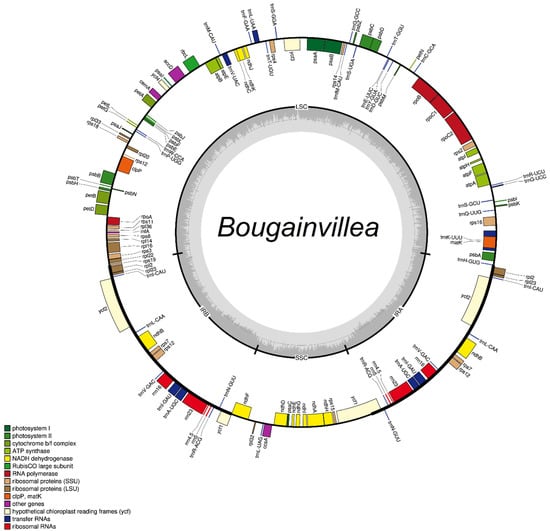The image is a detailed diagram set against a white background, featuring a central focus and intricate annotations. At the very center of the diagram, there is a light gray inner circle with the word "Bougainvillea" prominently displayed in black font. This inner circle is surrounded by a dark gray outer border, creating a sharp contrast. The border between the light and dark gray areas resembles an extremely fine, detailed bar graph.

Encircling this central area, there's an outer ring marked by a black line. Attached to this black line are numerous small, colored bar graph bars that extend both inside and outside of the circle. These bars vary in color, including green, red, blue, and yellow, and differ in size and shape, ranging from squares to rectangles. Each bar has writing next to it, providing specific details likely related to the colors.

In the lower left-hand corner of the frame, there is a color-coded guide, or key, that helps to interpret the colors of the different bars. This key lists various biochemicals, such as "photosystem 1" and "photosystem 2," corresponding to the different colored squares. The font used for the markings on the diagram is notably small and may be challenging to read.

Overall, the diagram appears to be a sophisticated visual representation, possibly related to biochemical data, with a focus on the different components surrounding the central theme of "Bougainvillea."